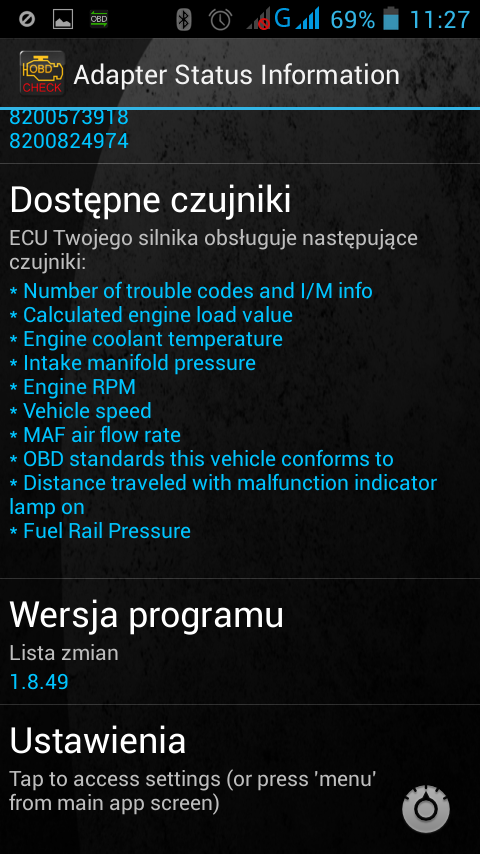The image is a rectangular screenshot from an Android cell phone, evident by the typical icons at the top such as signal bars, Bluetooth, battery percentage at 69%, and the time reading 11:27. The main content of the screenshot showcases the "Adapter Status Information" header in white text. To the left of this header is a distinctive yellow and red icon resembling a screw. Below the header are a series of long numbers and text in a foreign language, interspersed with English. 

The English text, formatted in a bulleted list with star symbols, details various vehicle diagnostics: number of trouble codes and IM info, calculated engine load value, engine coolant temperature, intake manifold pressure, engine RPM, vehicle speed, MAF airflow rate, OBD standards this vehicle conforms to, distance traveled with the malfunction indicator lamp on, and fuel rail pressure. Beneath this list is another section of text in the foreign language, followed by a prompt in white text stating, "Tap to access settings or press menu from main app screen." The background is black, highlighting the detailed information displayed prominently.